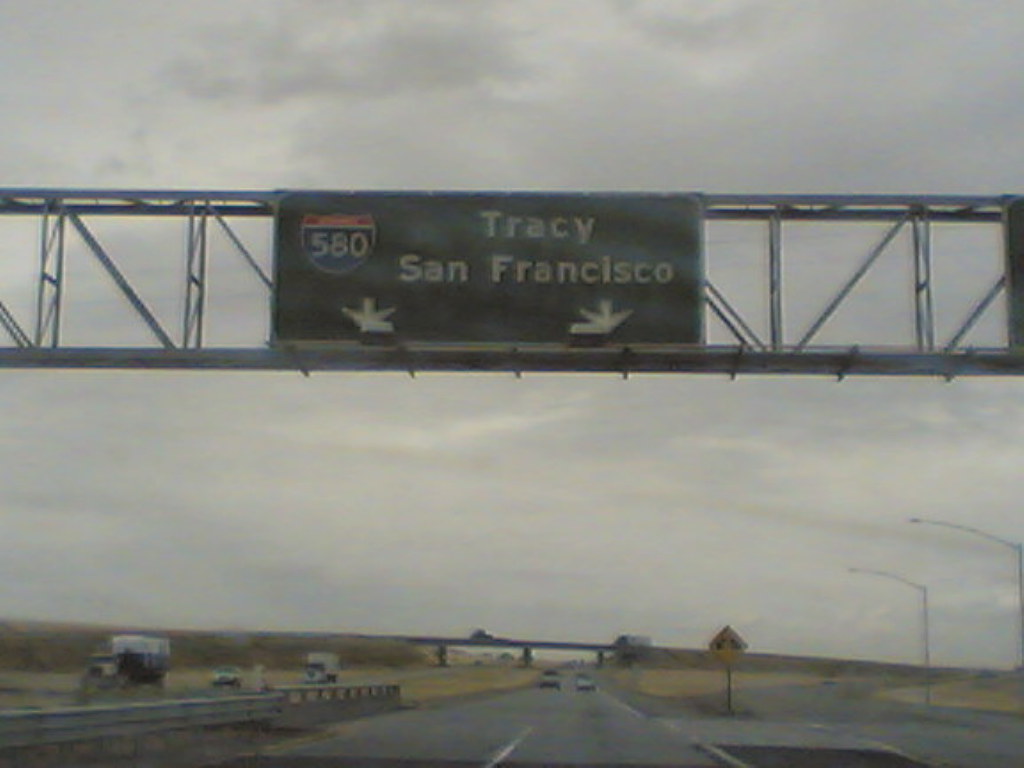This image captures a dreary daytime scene on Interstate Loop 580. The photo, likely taken with an older device, shows a gray, overcast sky suggestive of a winter day. The tanned patches of dead grass along the off-ramps, median, and both sides of the interstate reinforce the seasonal atmosphere. Prominently featured is an overhead sign supported by metal bars, which stretches across the highway. The sign directs drivers toward Tracy and San Francisco, with white text indicating the destinations and arrows pointing downward to guide lane selection. Additionally, a red, white, and blue highway shield displaying the number 580 is visible on the sign. In front of the vehicle, several cars and trucks are on the road, and further ahead is an overpass with a big truck nearing it. Street lights on the off-ramp are also seen, and on the opposite side of the highway, three vehicles approach, enhancing the sense of an active, albeit gloomy, travel day.